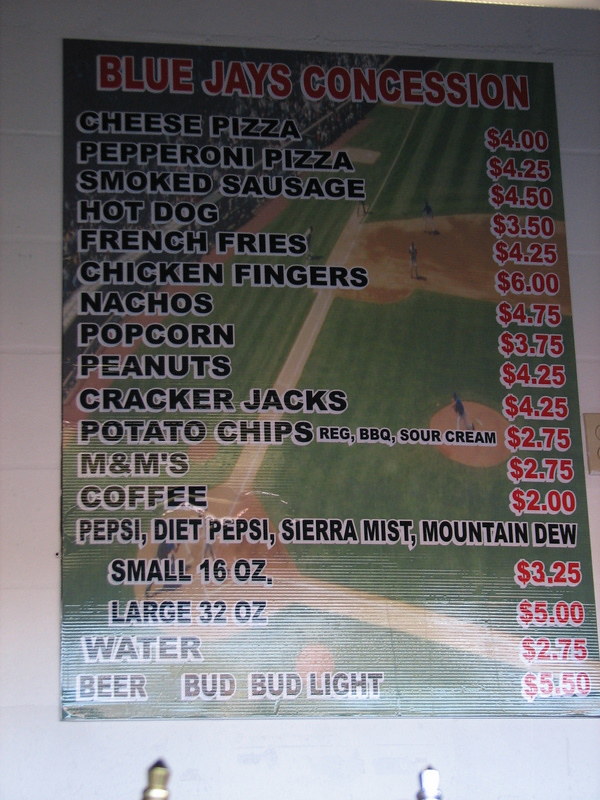This photograph captures a detailed menu from a concession stand, prominently displayed on a gray wall. The backdrop of the menu features a vibrant green baseball field, clearly depicting the infield, including third base, the pitcher's mound, and home plate. At the top of the menu, in striking red letters, it reads "Blue Jays Concession."

Beneath the header, the menu items are listed in black text, while the prices are highlighted in red. The offerings and their respective prices are as follows:

- Cheese Pizza: $4.00
- Pepperoni Pizza: $4.25
- Smoked Sausage: $4.50
- Hot Dog: $3.50
- French Fries: $4.25
- Chicken Fingers: $6.00
- Nachos: $4.75
- Popcorn: $3.75
- Peanuts: $4.25
- Cracker Jacks: $4.25
- Potato Chips (Regular, Barbecue, Sour Cream): $2.75
- M&Ms: $2.75
- Coffee: $2.00

The beverage options include:
- Pepsi, Diet Pepsi, Sierra Mist, Mountain Dew:
   - Small (16 oz): $3.25
   - Large (32 oz): $5.00
- Water: $2.75
- Beer (Bud and Bud Light): $5.50

The meticulously organized menu provides a comprehensive array of snacks and drinks, catering to a variety of tastes and preferences for visitors at the baseball field.